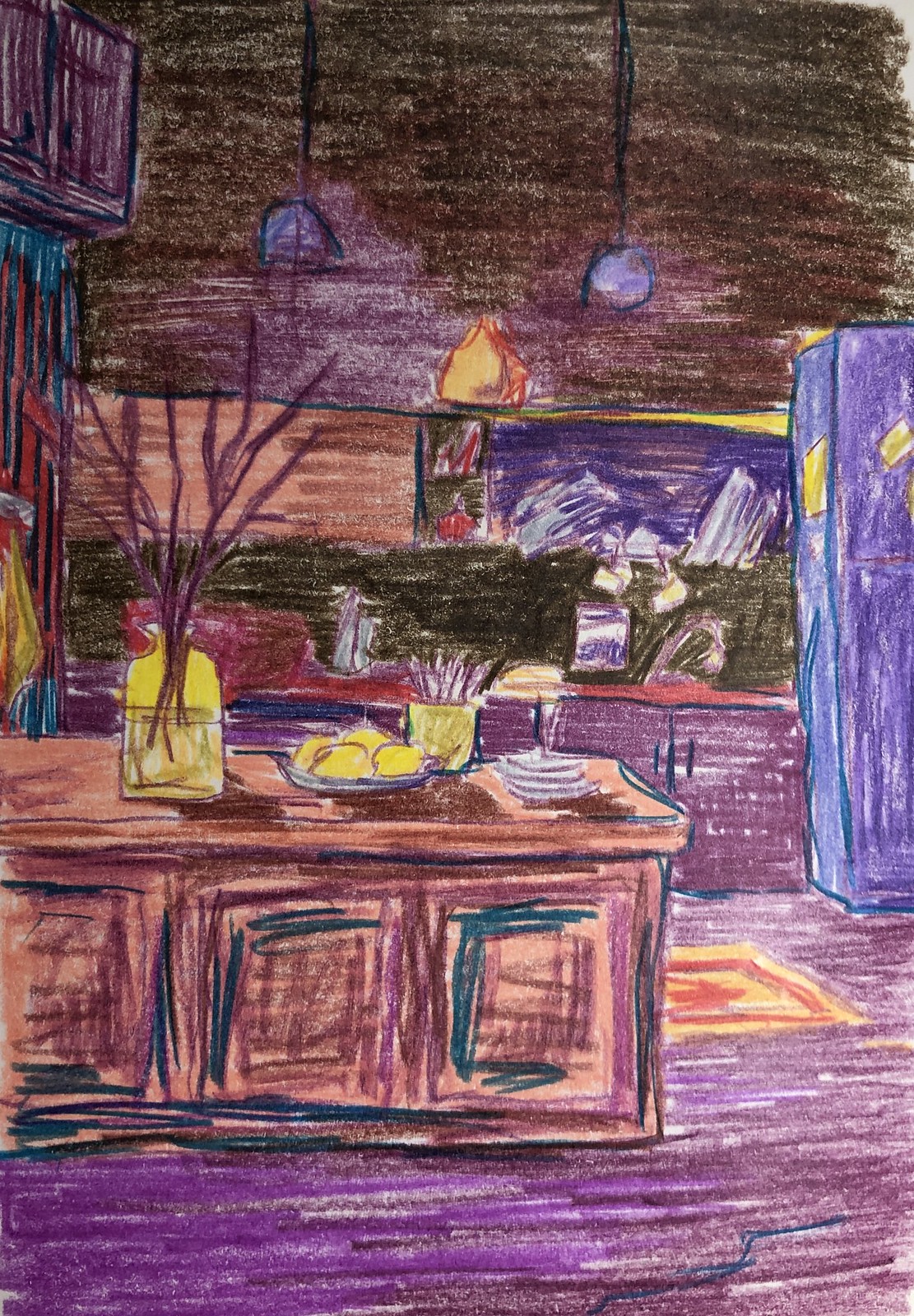This detailed hand-drawn piece of art appears to vividly illustrate the interior of a kitchen, created using colored pencil or possibly crayon. The image is dominated by hues of purple, creating a unique and imaginative atmosphere. The ceiling is notably dark, providing contrast to the rest of the scene, and is adorned with hanging lights featuring purple lampshades.

On the right side of the background, a refrigerator is discernible, adorned with several yellow items. To the left of the refrigerator, a window allows a view of what seems to be mountains, enhancing the sense of space within the room. Below the window, there is a countertop alongside a cupboard, potentially indicating the location of a sink.

As your eyes transition further left across the drawing, additional cupboards and countertops come into view, suggesting a well-equipped kitchen. The foreground is striking with its purple floor and a wooden countertop, which prominently features plates resting on its surface. Additionally, a transparent container with a yellowish tint, filled with branches, is also placed on the counter. A plate of sliced lemons adds a fresh, vibrant touch to the scene.

Overall, the art captures the essence of a cozy kitchen space, filled with rich details and a whimsical palette.